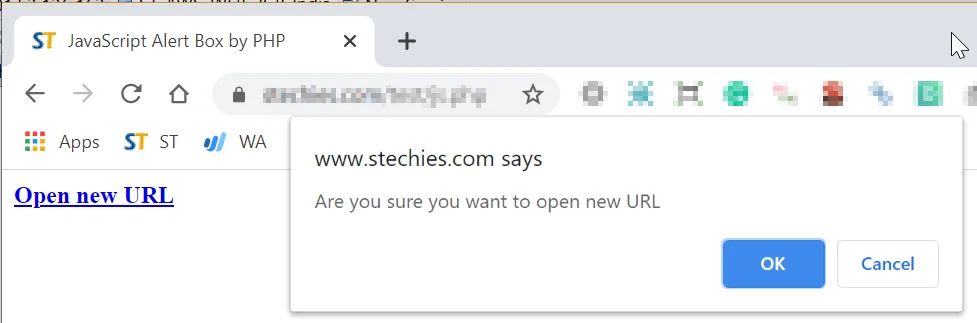This image depicts a webpage featuring a JavaScript alert box implemented with PHP. At the top, there's a web browser interface showing the letters "ST," where "S" is in blue and "T" is in gold. Just below the browser URL bar, there is a gray navigation bar. The content displayed appears intentionally skewed and blurry, offering a distorted view of the page elements. 

On the left side, there are navigation icons, including arrows and a home icon, whereas all icons on the right side are multi-colored (green, red, and gray) and also blurred. 

A prominent feature is a pop-up alert box from the site www.stetchies.com, with the question: "Are you sure you want to open a new URL?" The pop-up provides two options: a blue "OK" button and a white "Cancel" button.

Below this alert, the page shows a section styled in multicolored lettering reminiscent of Google's color scheme, labeled "Apps." There is also a clickable underlined link in blue reading "Open new URL" with blue curved lines adjacent to the text. 

At the top, there is an almost cut-off tan box with some indiscernible text, further contributing to the overall chaotic and unclear presentation of the web page.